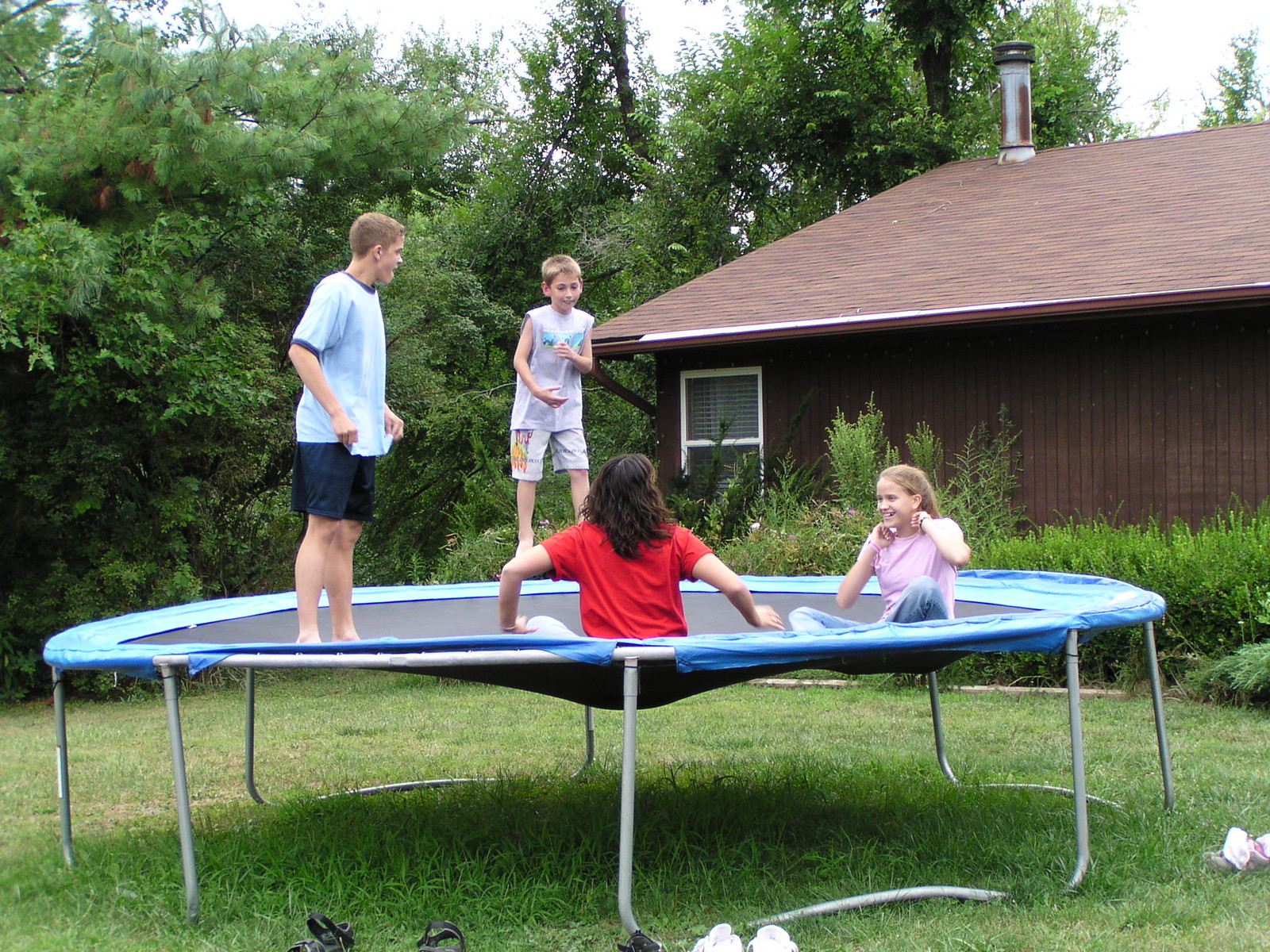In this photograph of a backyard scene, the sky is overcast with thick gray clouds, creating a bright yet somber afternoon atmosphere. The yard is enclosed by a dense collection of trees and bushes, their healthy green foliage providing seclusion. A dark brown, wooden house stands on the right, featuring light brown oil-based shingles on its pitched roof and a chimney, rusty on the sides, protruding from the top. The house has a white-framed window on the left side, and is bordered by neatly trimmed shrubs.

The centerpiece of the yard is a trampoline with metal legs, standing about three feet off the ground. Surrounding its edge is a blue fabric cover, with a black jumping surface sagging slightly, perhaps due to age or the weight of the occupants. Four children are on the trampoline: two boys stand up and face each other, while two girls sit crisscross applesauce, laughing together. The boy on the left, with short blonde hair, wears dark blue shorts and a matching t-shirt. The boy on the right, with closely-cropped blonde hair, dons tan shorts and a gray sleeveless t-shirt. One girl, a brunette with a red t-shirt, has her back to the viewer as she looks at the other girl, who wears blue jeans and a pink shirt, her long blonde hair framing her smiling face. Scattered in the grass around the trampoline are various shoes and sandals, left behind by the children.